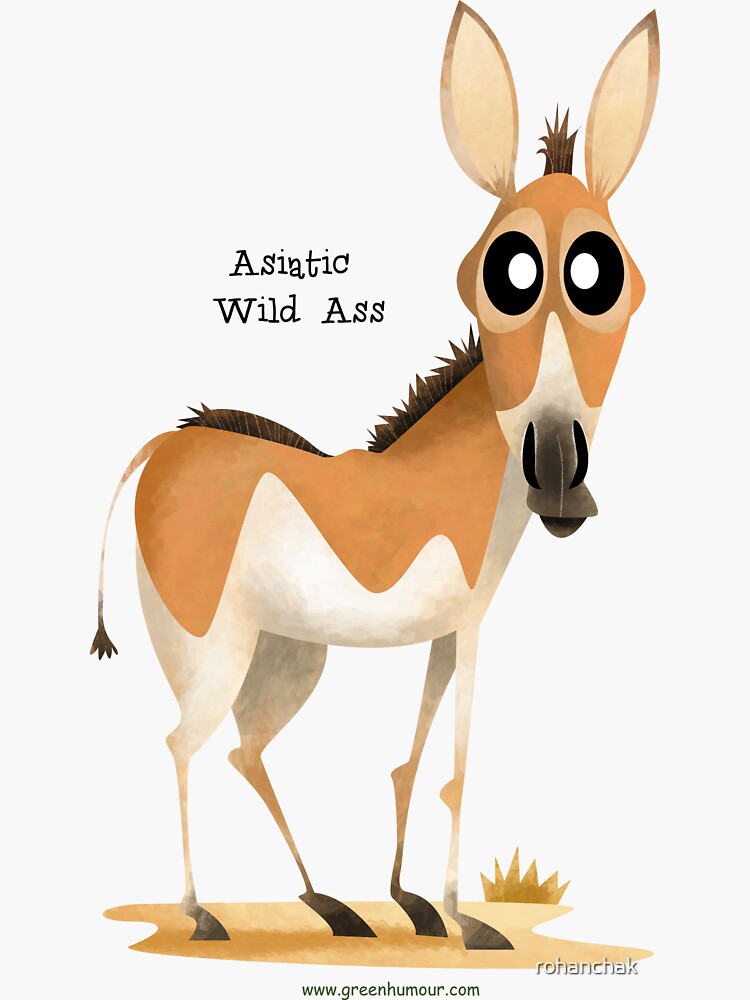The image is a detailed, cartoon-style drawing with slightly exaggerated features, presenting a humorous depiction of an animal that resembles a donkey or horse. The scene is set against a flat white background with the animal standing on a small patch of barren, sand-colored ground, highlighted with some textures to give it depth and shadow, resembling a desert or African setting. The animal, identified as an "Asiatic Wild Ass" in the text above it, has a tan body with large, sad, bewildered black eyes and a mouth colored in dark hues. It possesses a very small tail, brown hooves, and some hair on its back, adding to its slightly exaggerated appearance. Additionally, a small piece of desert grass can be seen behind the animal, textured and highlighted to enhance the scene. The illustration also includes text indicating its humorous nature with the phrase "ASCIDIC WILD ASS" followed by the website "www.greenhumor.com" and a copyright note for artist Rohan Chak.